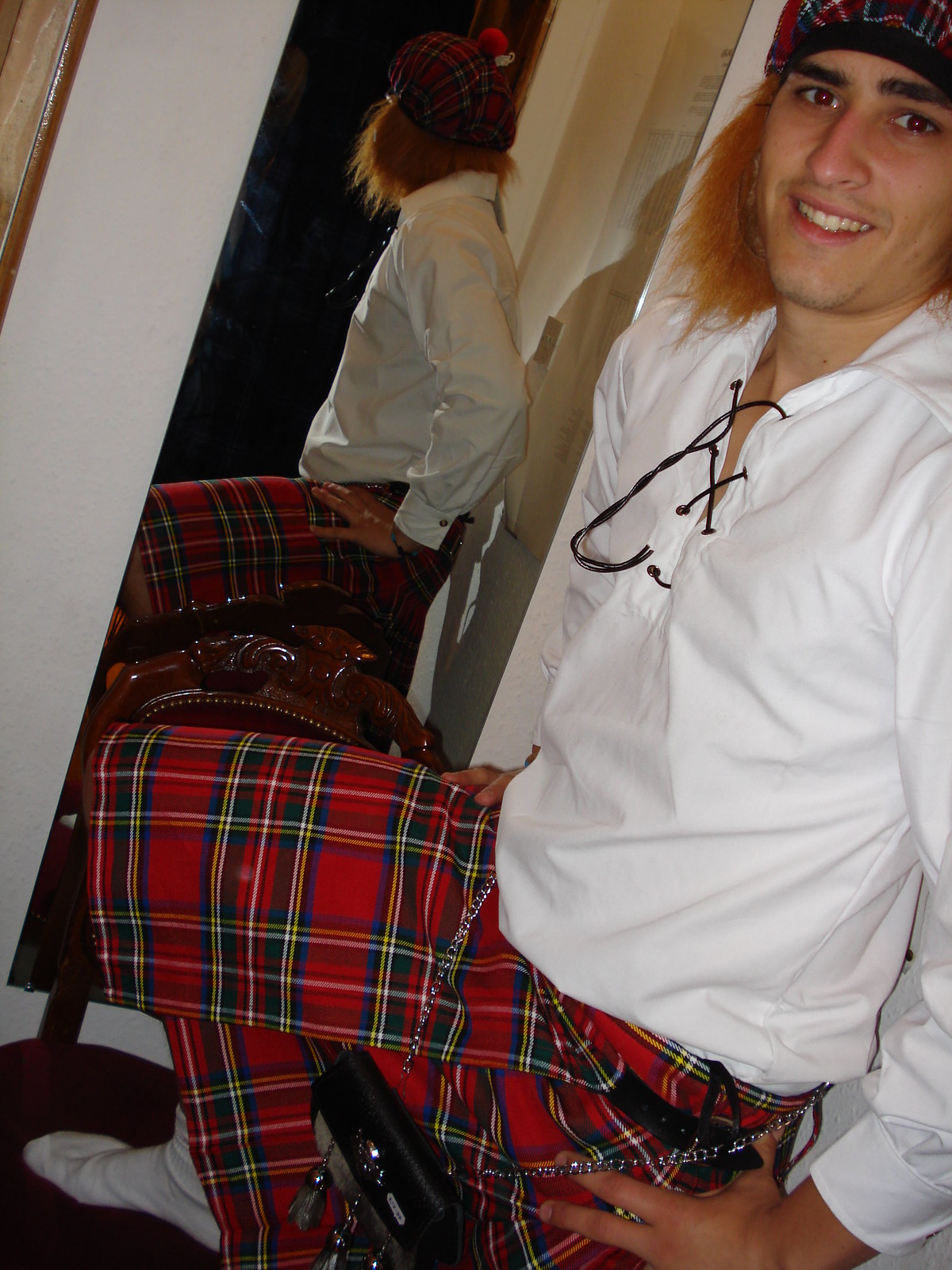This photograph depicts a man dressed in traditional Scottish attire. He is situated on the right side of the image, prominently covering the front right area. The man is squatting or possibly sitting in an L-shaped pose, with his head higher and further to the right than his midsection. He is wearing a red tartan kilt, adorned with hints of green, yellow, and other colors, paired with a sporran—the tasseled pouch hanging in front. His outfit includes a white long-sleeved shirt fastened at the collar with a dark cord, and he has a silver chain around his waist. The man has thick black eyebrows, light reddish hair, and a matching tartan tam-o-shanter with a red ball on top. His right leg is propped up on a dark wooden chair, revealing a white sock. Behind him, a tall, rectangular vertical mirror reflects his image, showing the back of his head, his right arm, which is placed on his hip, and his right leg, which are not visible in the main perspective. He gazes at the camera with a proud expression, smiling broadly. The mirror is positioned at an angle, with the bottom further to the left than the top, providing a full view of his confident stance.